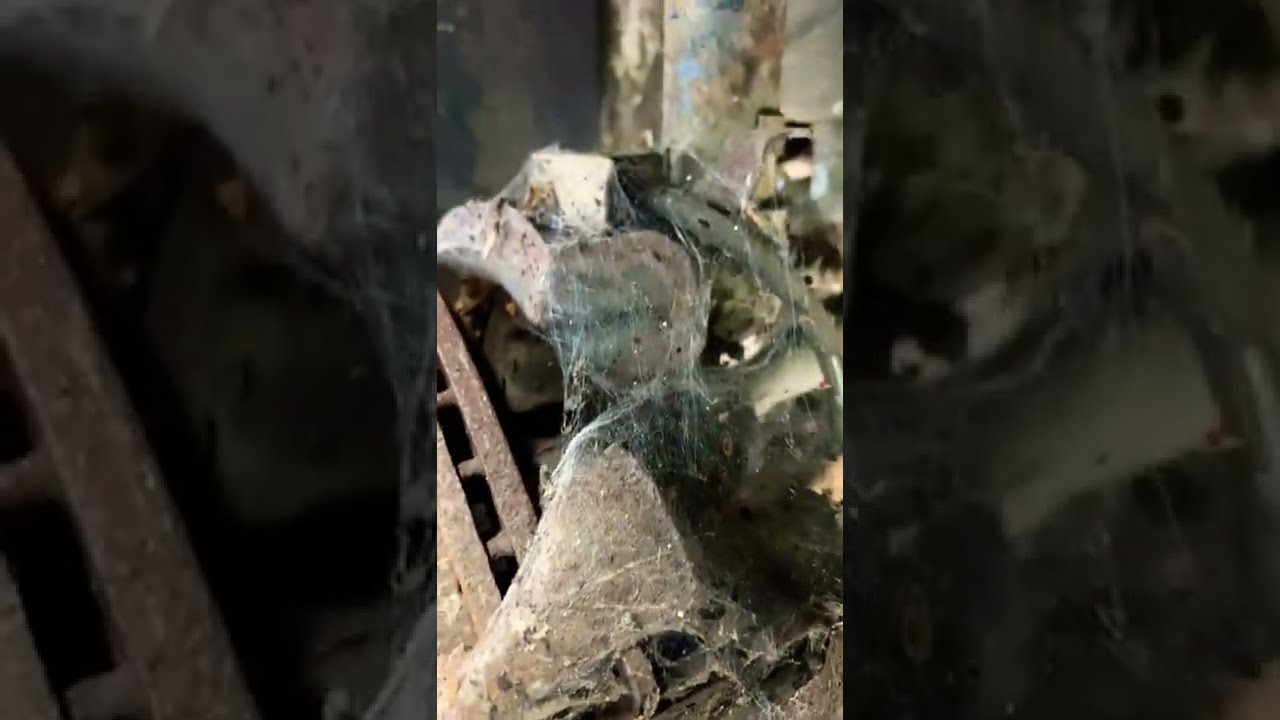The photograph captures a close-up view of an old, rusted metallic machine, which is outdoors, divided into three vertical sections. The left and right sections are darkened close-ups, highlighting the central part of the image where the machine is located. This dilapidated device is heavily corroded, covered in spider webs and cobwebs, making it appear brown and heavily weathered. It features a pipe and parts that resemble a mechanical hand with two finger-like extensions, indicating it might be a part of some neglected machinery that hasn't been used in a long time. The background reveals faint details of a dirty wall, a street, or curb with some visible blue markings, and a bit of water, suggesting an outdoor setting. The overall color palette is dominated by rust tones, silvers, blacks, browns, and some blues, set against a backdrop of dirt and grime. The image is taken during the day, offering clear visibility of the deteriorated state of the machine.